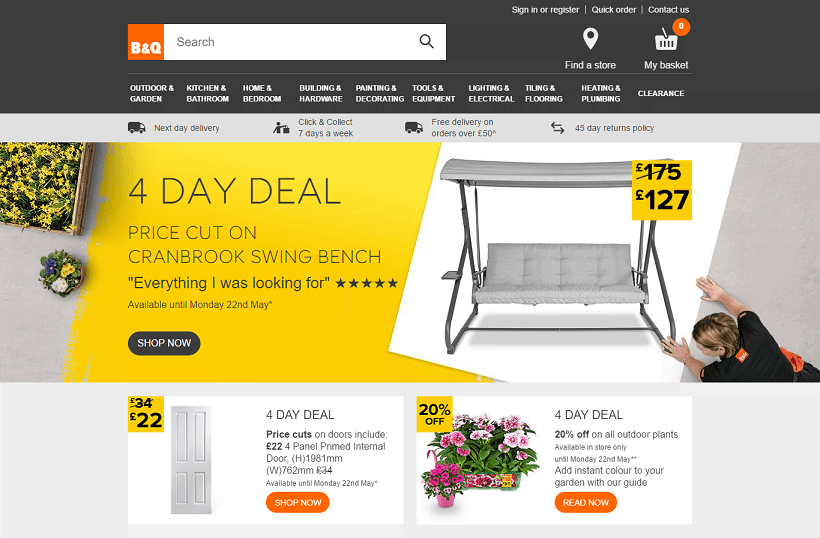The screenshot displays a home goods retailer website, identified by the B&Q logo in orange located in the top corner beside a search window. The site offers 10 different sort options beneath the search bar, with categories including outdoor and garden to clearance. Immediately below this segment, a small menu bar highlights features such as next-day delivery, click and collect available seven days a week, free delivery on orders over $50, and a 45-day returns policy.

The main section of the webpage is dominated by a bold yellow banner with large text announcing a "Four-Day Deal" featuring a price cut on the Cranbrook Swing Bench. A highlighted customer review below the text reads, "Everything I was looking for," accompanied by a five-star rating. The availability of this offer is clearly stated as valid until Monday, the 22nd of May. A small, black oval "Shop Now" button is positioned beneath this information.

To the right of this banner, an image of the Cranbrook Swing Bench shows it as a self-supporting structure with a swinging, sofa-like bench and an integrated canopy. A smaller yellow price box reveals the discounted price—from $175 to $127. In the lower right-hand corner of the screen, a person in a black shirt with orange accents appears to be whimsically arranging the photo of the swing bench.

Below the main deal, promotions for additional four-day deals are visible. One such deal features a white door priced at $22, reduced from $34. Another promotion offers a 20% discount on all outdoor plants, accompanied by a vibrant image of various plants.